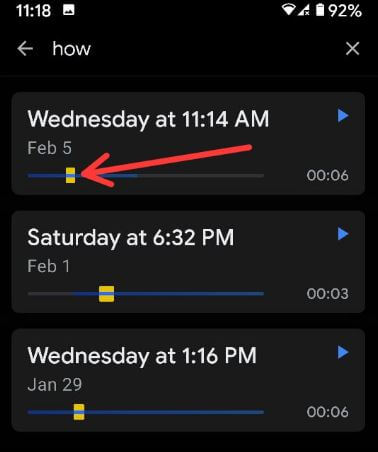This image is a screenshot from a smartphone displaying a list of voice memo recordings. The voice memos are arranged in descending order by date and time, with the most recent recording at the top. Specifically, the top entry is a memo from Wednesday, February 5th at 11:14 AM, followed by another from Saturday, February 1st at 6:32 PM, and an additional one from Wednesday, January 29th at 1:16 PM. Each memo features a progress bar with a red toggle, allowing the user to navigate to specific timestamps within the recording. A red arrow points to this toggle, highlighting its location. Each entry also includes options to play the recording and displays the timestamp corresponding to the position of the toggle on the progress bar.